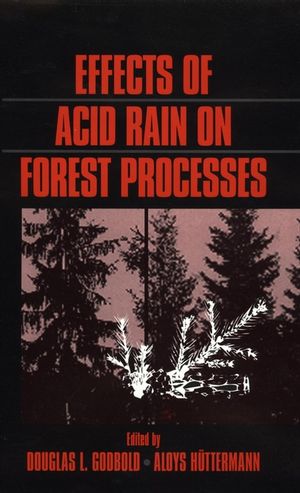The cover of the book "Effects of Acid Rain on Forest Processes," edited by Douglas L. Godbold and Alois Hüttermann, prominently features a tall, rectangular black background. The title, written in bold red capitalized block letters, is displayed across two horizontal lines near the top. Beneath the title, there's a detailed illustration: a beige box containing a depiction of dark, almost black evergreen trees and contrasting white shapes, simulating branches seemingly damage by acid rain. The illustration is bisected by a vertical black line, visually representing the dichotomy between the untouched and affected forest. The editor's names are listed at the bottom in the same red lettering. The overall composition gives a dramatic and somber representation of the detrimental effects of acid rain on forest ecosystems.